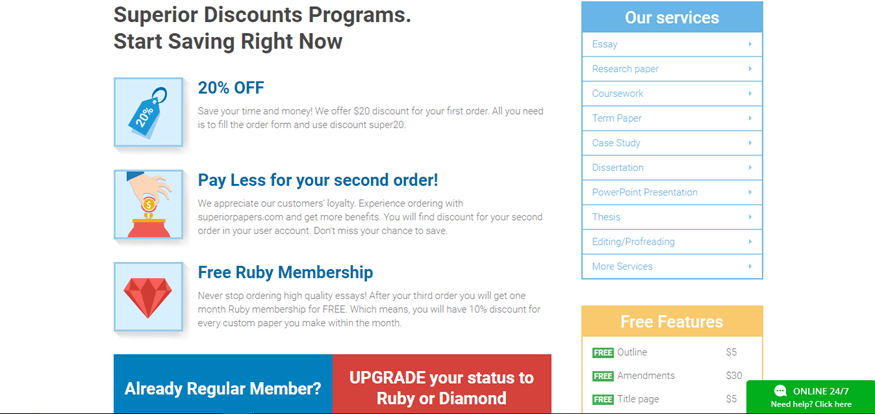**Superior Discount Programs - Start Saving Now!**

On the left side of the image, there are three icons accompanied by detailed discount information:

1. **20% Off Tag Icon**: 
   - **Caption**: "Save Your Time and Money"
   - **Details**: "We offer a $20 discount on your first order. Simply fill in the order form and use the discount code 'SUPER20'."

2. **Coin into Bag Icon**:
   - **Caption**: "Pay Less for Your Second Order"
   - **Details**: "We appreciate our customers' loyalty. Experience ordering with SuperPapers.com and gain more benefits. The discount for your second order can be found in your user account. Don’t miss your chance to save!"

3. **Diamond Icon**:
   - **Caption**: "Free Ruby Membership"
   - **Details**: "Never stop ordering high-quality essays. After your third order, you will receive one month of Ruby Membership for free, entitling you to a 10% discount on every custom paper you order within that month. 
   - **Question**: "Already a member?"
   - **Option**: "Upgrade your status to Ruby or Diamond."

On the right side of the image, there's a table listing the various services and features provided:

- **Our Services**:
  - Essay
  - Research Paper
  - Course Work
  - Term Paper
  - Case Study
  - Dissertation
  - PowerPoint Presentation
  - Additional Editorial Services under "Editing Pro"

- **Free Features**:
  - Outline: $35 value
  - Amendments: $30 value
  - Title Page: $5 value

These programs and features aim to provide significant value and savings to customers while ensuring access to high-quality academic assistance.